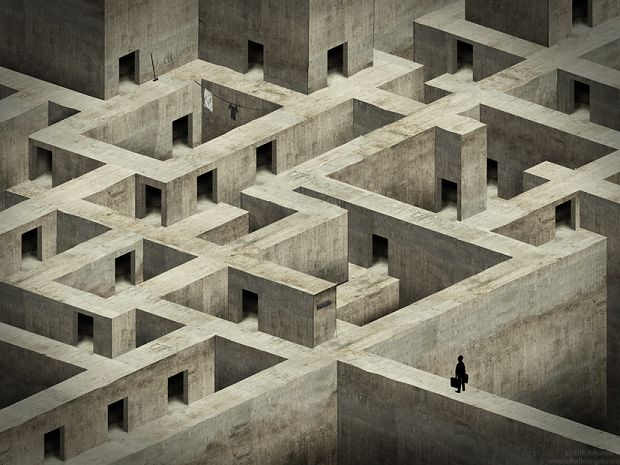In this surreal, monochromatic illustration, a small, silhouetted man stands on a narrow stone wall at the lower left of the image, holding briefcases in both hands. He gazes into a disorienting, labyrinthine structure made entirely of cement blocks and dark doorways. The scene evokes the optical illusions of an Escher staircase, where angular, overlapping planes create a confusing maze. Each door seems to lead to an impossible destination, enhancing the sense of an urban maze built from stark, straight-lined walls. The more you look, the more the stone pathways defy logical navigation, deepening the trippy, surreal quality of the artwork. The overall background is very dark, further emphasizing the silhouette and the intricate, baffling maze before him.